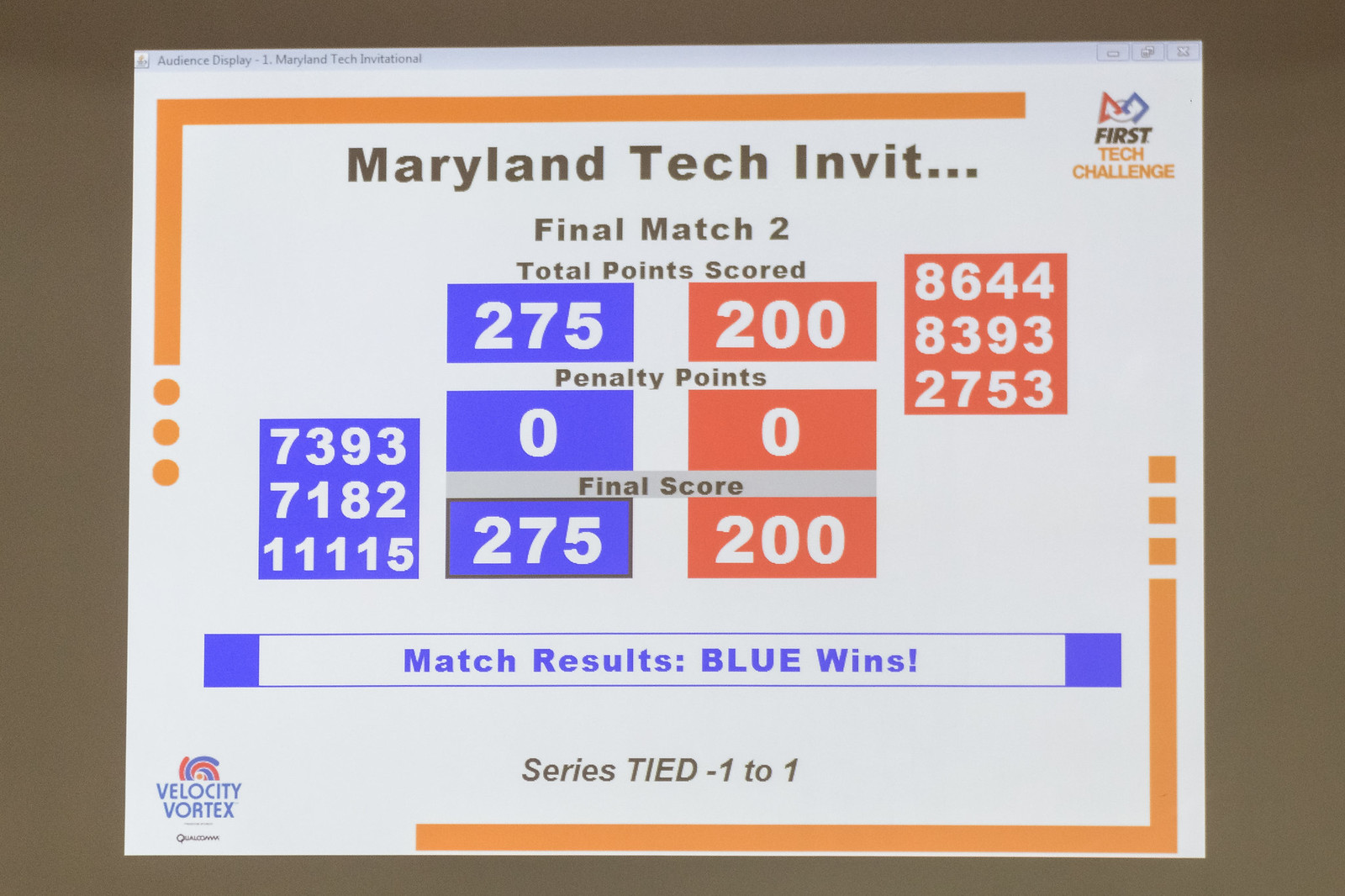The image displays an LED screen showing the "Maryland Tech Invitational" with a detailed match summary. At the top, within an orange-bordered section labeled "Audience Display," the text reads: "Maryland Tech Invit..." followed by "Final Match 2". Below, "Total Points Scored" is listed, with the blue side scoring 275 points and the red side scoring 200 points. "Penalty Points" for both sides are zero. The "Final Score" mirrors the total points, confirming the blue side leads with 275 over the red side's 200. The "Match Results" indicate "Blue Wins," and the series is "Tied 1 to 1". The screen's design includes various orange elements: three orange scores on the right and three orange circles on the left. The company logo, "Velocity Vortex," is located at the bottom left, while "First Tech Challenge" is noted at the top right.